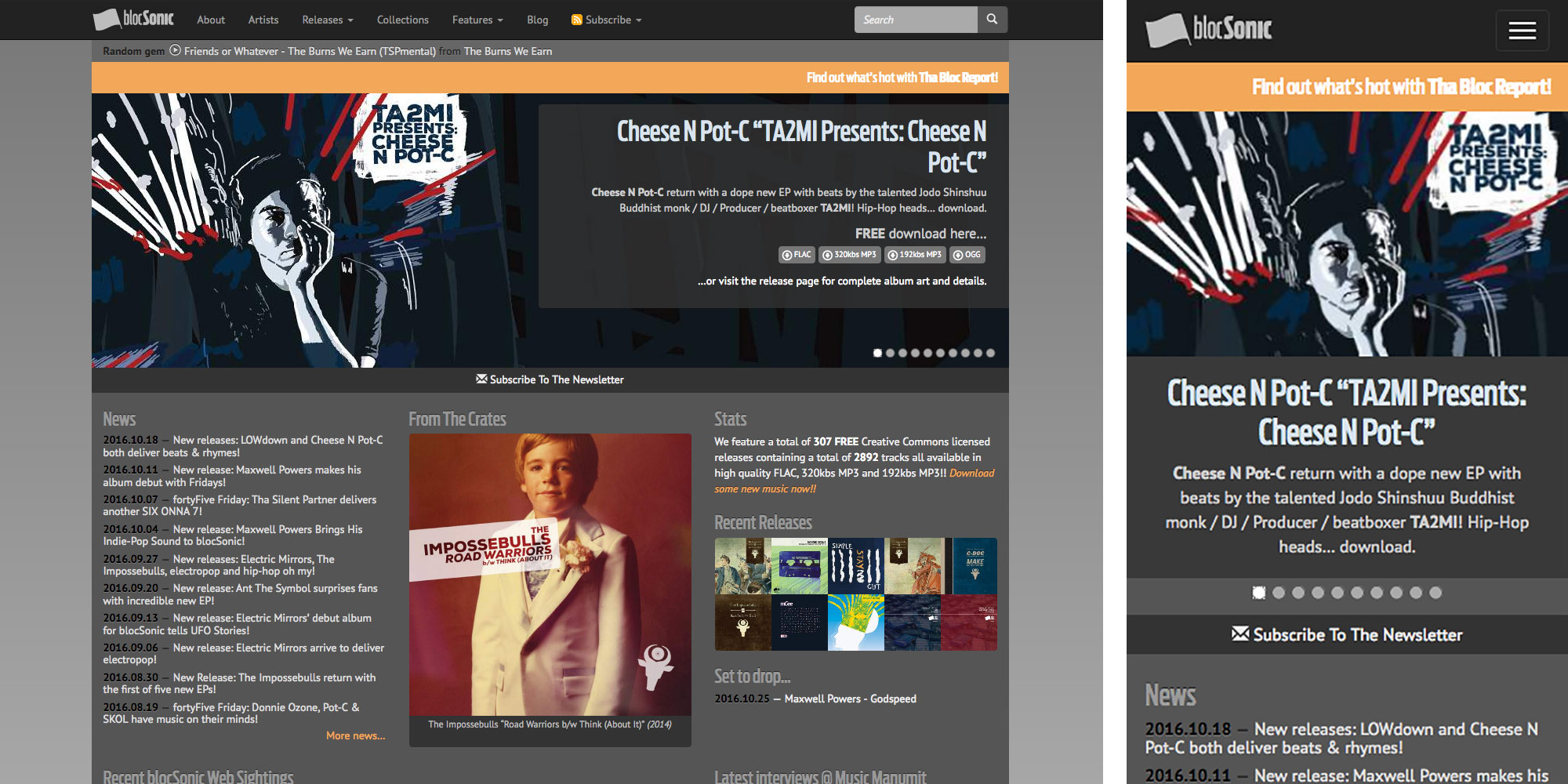This image showcases a website designed for a dark mode interface, displaying both desktop and mobile app experiences. At the top of the desktop layout, there's a logo featuring a flag with the text "Block Sonic." The navigation menu includes options such as About, Articles, Features, Blog, Subscribe, and a search box positioned on the right-hand side. 

For the mobile app, still displaying the "Block Sonic" logo, three horizontal lines signify a dropdown menu. Both experiences feature an eye-catching orange banner that encourages users to "find out what's hot with Block Report."

Central to the design is a stylized illustration of a man, predominantly cast in shadow, suggesting he is likely Caucasian. He rests his head in his right hand with his elbow on a table. Above him, a speech bubble reads, "TA2MI presents Cheese and Pot-C," and white and red lines emanate from the character, resembling either energy or exclamation marks.

Beneath this illustration, a section lists news items by date, providing users with the latest updates and information in a chronological format.